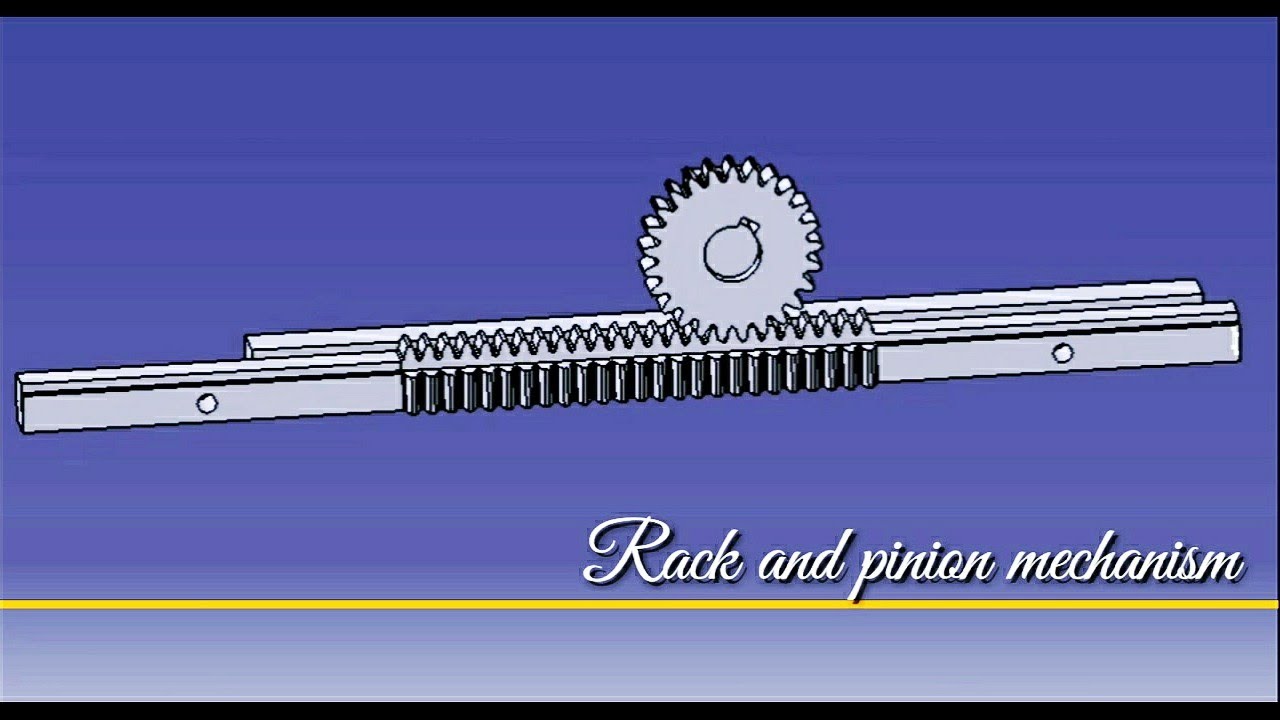The image features a stylized illustration resembling an advertisement, showcasing a rack and pinion mechanism prominently. The design appears in a pen and ink drawing style, possibly enhanced with a computer graphic program, giving it a detailed, sketch-like appearance. The mechanism includes a silver-colored cogwheel meshing with a metal bar that has teeth and two screw holes, suggesting it might originate from a technical or automotive manual. Behind this bar, there's another metal rod without teeth. The background gradient transitions from a deep purple at the top to a lighter lavender at the bottom, framing the mechanism in an attractive color scheme. The image has a black border, adding to its presentation. Above a yellow bar that runs across the lower part of the image, there is cursive text saying "rack and pinion mechanism." This indicates its purpose as possibly part of a larger sequence of instructional or promotional visuals.